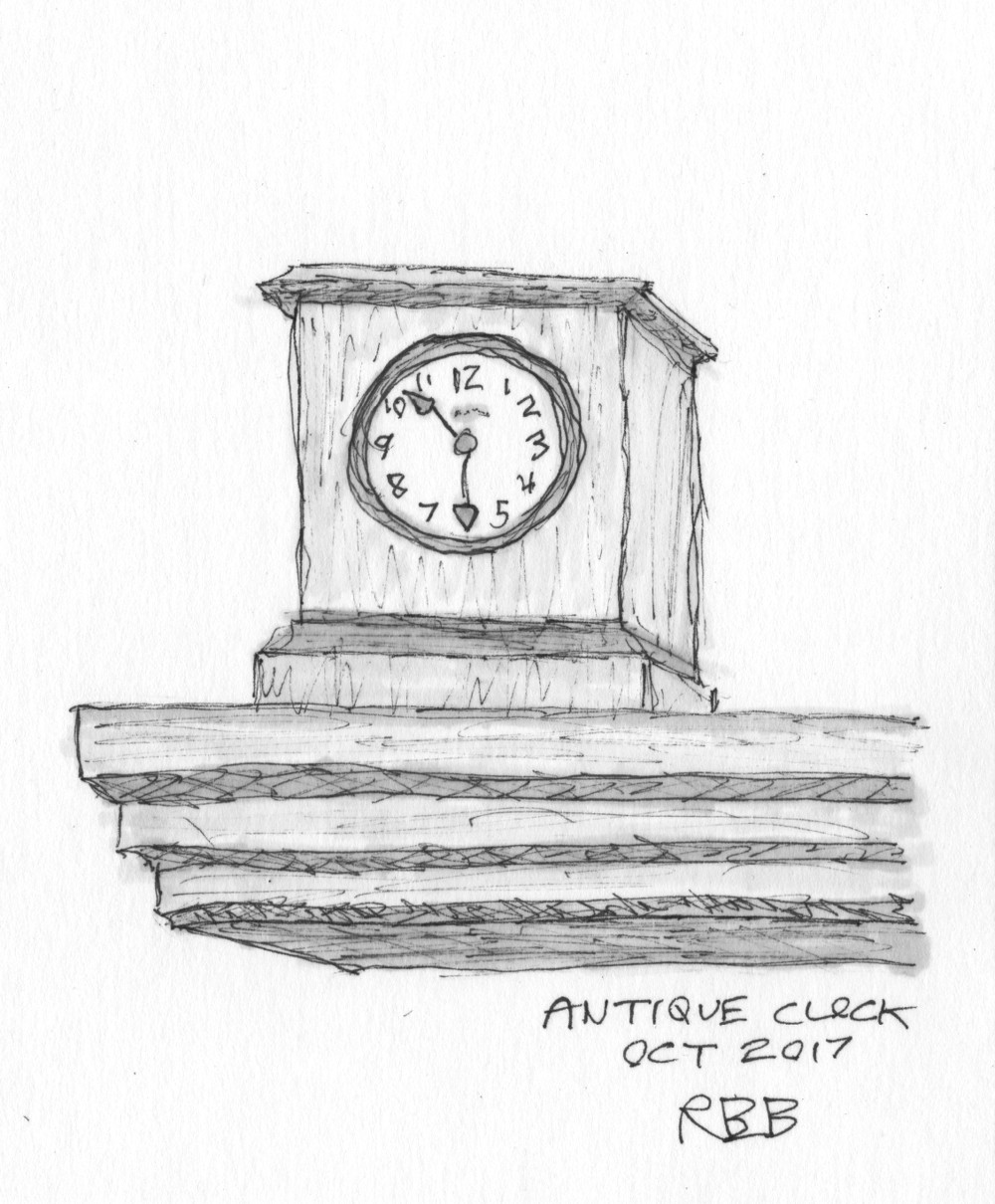This detailed pencil drawing depicts a square-shaped mantle clock with a circular clock face set against a darker gray background. The clock face features numbers from 1 to 12, with the minute hand positioned over the 6 and the hour hand between the 10 and 11, giving the time as approximately 5:52. The sketch shows an intricate design, with the clock housed on a three-tiered wooden shelf. Each tier is carefully shaded in varying tones of gray, with the topmost tier highlighted by a lighter gray roof and darker edges. The middle tier appears lighter in tone, while the base is drawn with darker shading. The artist's attention to detail is evident in the rough, textured lines that give depth to the clock and the shelf. In the bottom right corner, the words "Antique Clock, Oct. 2017, RBB" are inscribed in black ink, with the artist's initials featuring a distinctive line through both B's. The background of the drawing remains clean and white, emphasizing the meticulous craftsmanship of the clock and its supporting structure.